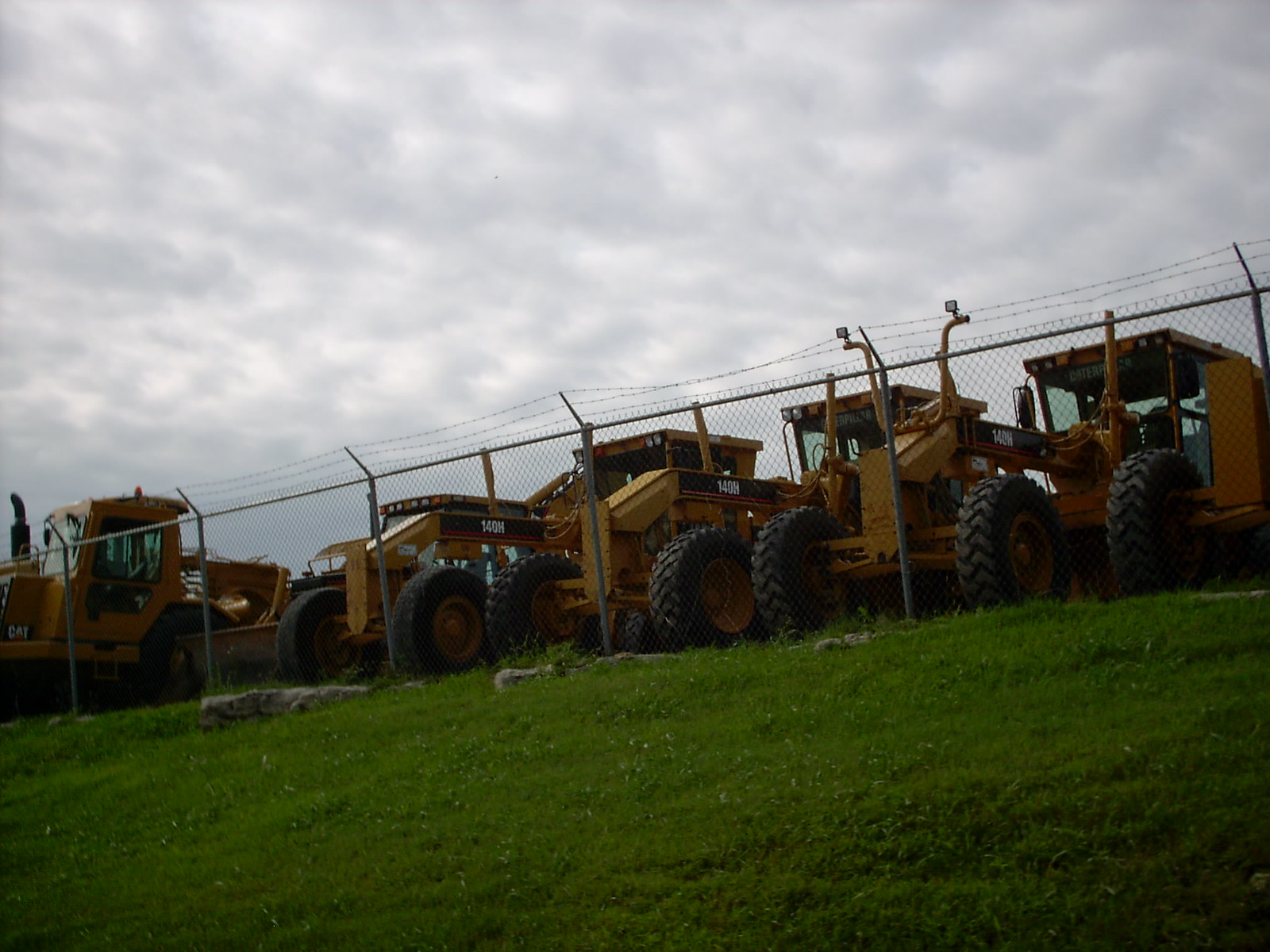In the image set outdoors, the sky is filled with unbroken rows of puffy white clouds, highlighted in parts by the sun behind them. In the foreground, a lush, green, grassy hill dotted with tiny white daisies is visible. There are a few large rocks scattered on the grass. A chain-link fence topped with a bracket and three lines of barbed wire secures the area on the hillside. Beyond this safety fencing, several pieces of bright yellow heavy machinery—likely made by Caterpillar—are lined up. These include various types of equipment such as bulldozers, all featuring large black tires of varying sizes. Each piece of machinery has lights atop the driver's area, with some sporting square lights while others have different lighting configurations.